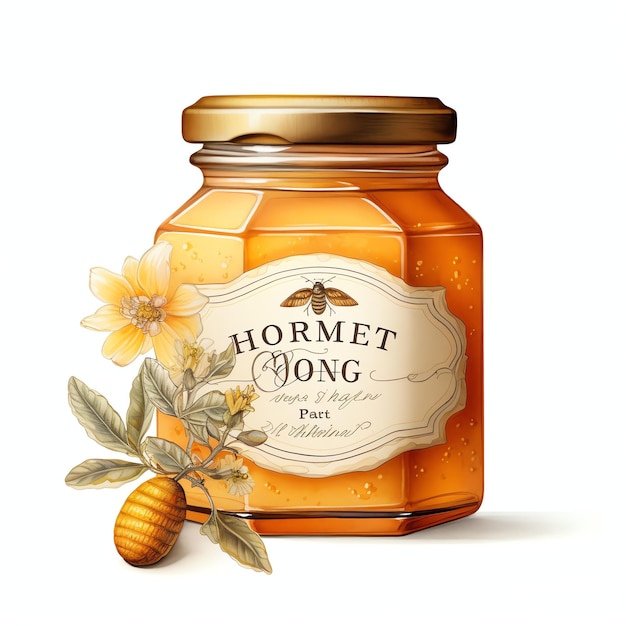This digital or AI-generated image features an artistic rendition of a hexagonal jar of honey with a golden lid, exuding a rich golden-amber hue illuminated beautifully within its glass container. The jar bears an off-white, oval-ish paper label with a prominent 'B' and the text "HORMETONG, O-N-G, PART," along with some indistinct cursive script. Arrayed in front of the jar, to the left, lies a delicate still life of yellow, light-colored flowers, and pale gray-green leaves. Additionally, a golden, egg-shaped orb decorated with horizontal bars is situated nearby, all resting against a blank white background. The image also depicts intricate details like the leaves sprouting from what appears to be a nut at the base, enhancing the natural essence captured in the artwork.